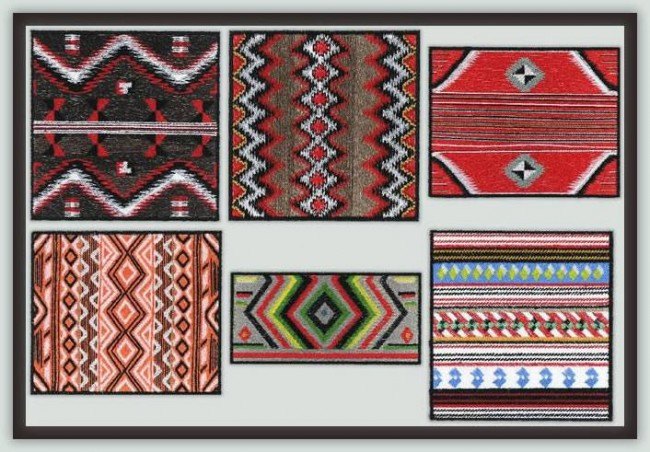The image depicts a detailed display of six framed rugs, each with unique Native American-inspired patterns and vibrant colors. These rugs are meticulously arranged against a plain white mat and encased in brown borders, giving them a polished and museum-like presentation. Each rug is rectangular or square, featuring an array of zigzag and diamond motifs.

The top left rug stands out with its black, red, and white zigzag pattern, with black serving as the background. Beneath it, the bottom left rug features a striking brown and pink combination, highlighted by brown zigzags and pink triangular and diamond shapes. 

Moving to the middle row, the top middle rug is adorned in a red, white, black, and gray vertical zigzag pattern, while the middle bottom rug introduces a new palette of green, red, black, yellow, and gray, full of intricate diamond designs. 

The top right rug predominantly showcases red hues, complemented by gray, white, and black patterns, while the bottom right adds a hint of blue to its Native American-inspired design, reminiscent of Southwestern craftsmanship.

Overall, the rugs exemplify a variety of traditional patterns and colors, creating a visually striking and culturally rich display.